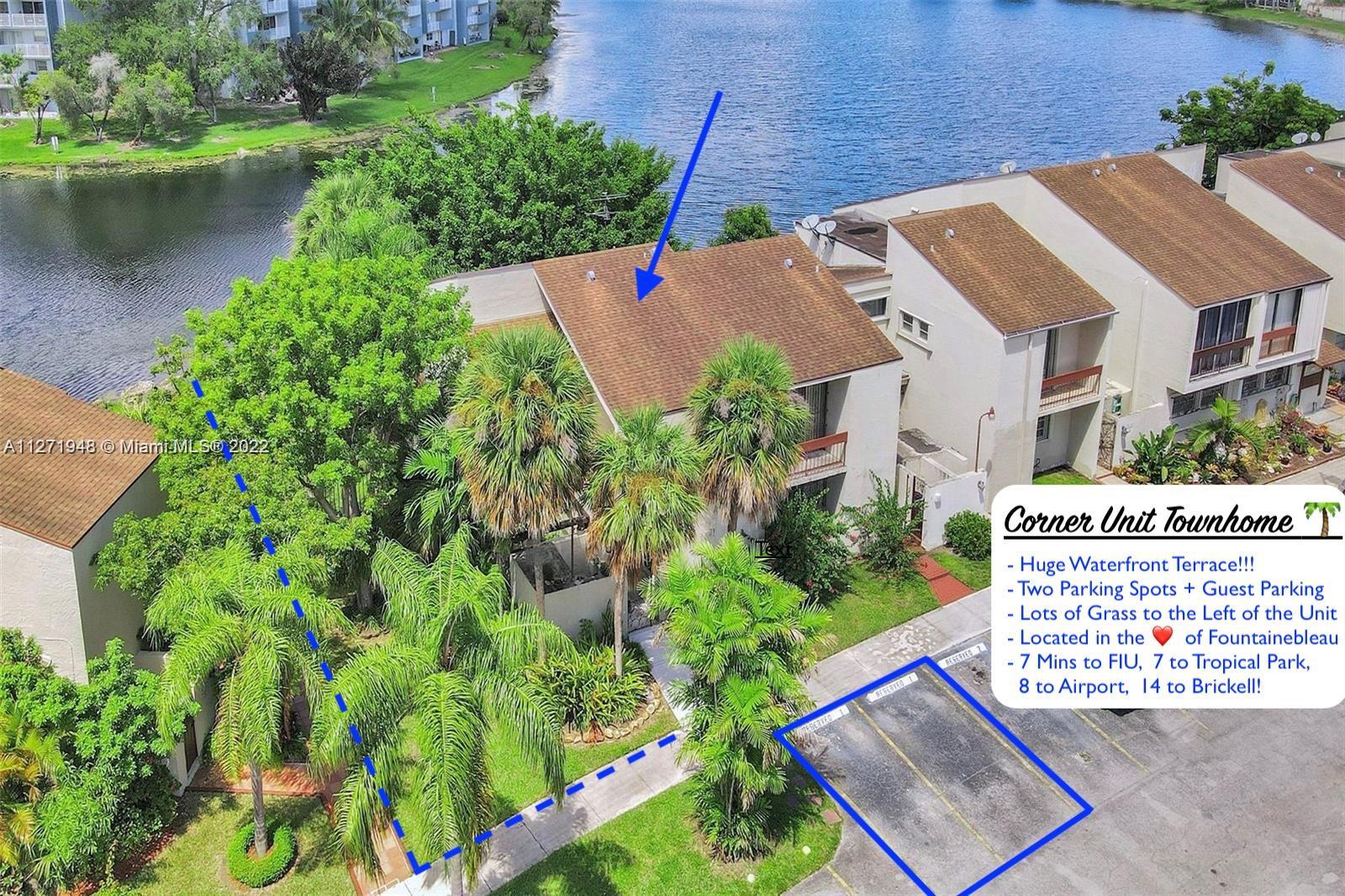This image is a detailed aerial photograph showcasing a corner unit townhouse located in the heart of Fountain Blue. The scene features a large body of blue water with ripples, reflecting the surroundings. The property, outlined by a white border, includes a huge waterfront terrace, ample grass area to the left, and two designated parking spots in a large shared parking lot. Additional guest parking is available. The view also includes marked sidewalks, various houses, and apartment buildings within the vicinity. Notably, from the townhome, it's a seven-minute drive to FIU, another seven to Tropical Park, eight minutes to the airport, and 14 minutes to Brickell. The bottom right of the image showcases essential listing details outlined in white text.